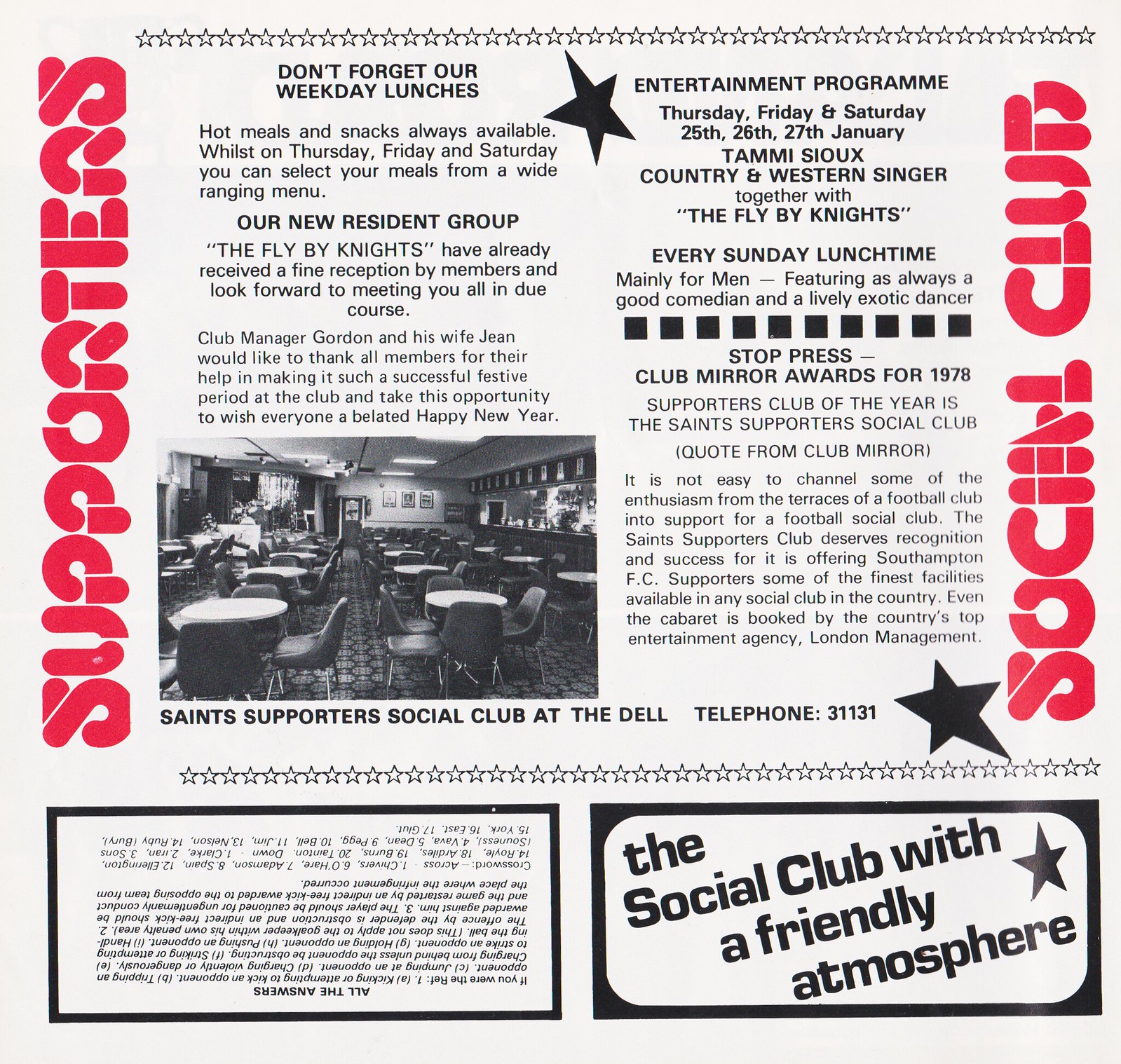The image displays an antique flyer for the Supporters Social Club, prominently featuring red, white, and black colors, along with various shades of grey. The layout includes centered imagery of the club's interior, showing tables, chairs, and a bar to the right, indicative of a restaurant setting. In red letters, "Supporters" is vertically written on the left, while "Social Club" appears on the right, both framed by a line of stars. The flyer boasts details about weekday lunches, highlighting that hot meals and snacks are always available. It features an entertainment program for Thursday, Friday, and Saturday, from 25th to 27th January, including performances by Tammy Sue, a country and western singer, and the resident group, the Flyby Knights. An additional paragraph promotes the club's friendly atmosphere, emphasizing events such as country singing on Sundays and a program mainly for men, complete with comedian acts and an exotic dancer. The bottom of the flyer also hints at a trivia or crossword puzzle section, adding to the vintage charm of the document.